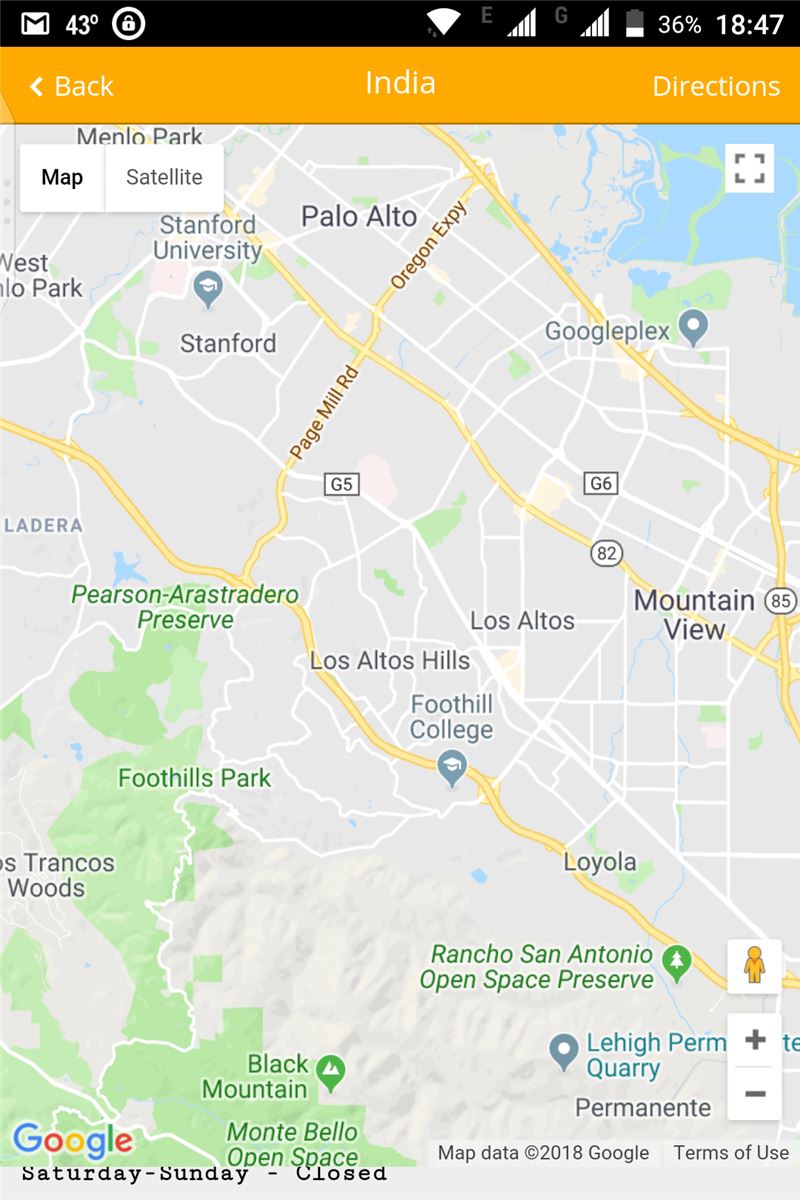**Detailed Description of a Google Maps Screenshot:**

The image is a screenshot of a Google Maps interface captured on a smartphone. The topmost part of the screen, the status bar, has a black background with white text and icons. In the upper left corner, there's a Gmail notification icon followed by the current temperature, 43 degrees Fahrenheit. Beside it is a lock icon. On the right side of the status bar, there are signal bars whose exact purpose is unclear, along with a battery icon indicating a 36% charge, which is also repeated in text. The current time displayed is 18:47.

The map itself is labelled with a top banner indicating the location as "India" in white text against an orange background, even though the map displayed is actually of California. On the left side of this banner is a 'Back' button, also in white text, and on the right side is a 'Directions' button, again in white text.

The main content of the image focuses on a detailed map of the Palo Alto area in California. Prominent labels include "Palo Alto," "Stanford University," "Googleplex," and nearby locations such as "Los Altos Hills," "Foothill College," "Mountain View," "Rancho San Antonio Open Space Preserve," "Black Mountain," and "Montebello Open Space."

The map is filled with various geographical markers outlining well-known institutions, natural reserves, and other significant areas within the surrounding Palo Alto and greater Silicon Valley region.